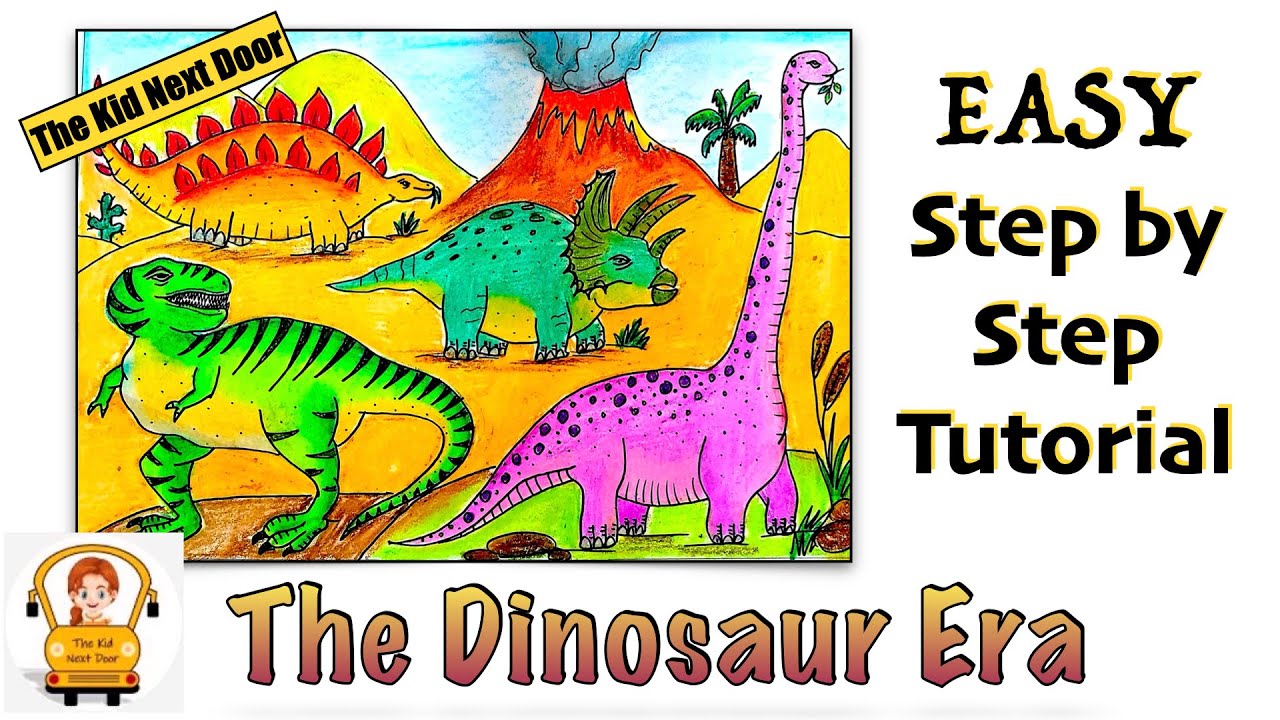This computer-generated cartoon image promotes a tutorial and features a colorful prehistoric landscape. Central to the image is a bordered square depicting a vibrant scene with dinosaurs and a volcano. The dinosaurs include a purple long-necked dinosaur with black spots, a green Tyrannosaurus rex with black zebra-like stripes, a blue-green Stegosaurus with large horns, and a smaller, yellow dinosaur with red spikes. The background shows a red volcano emitting smoke against a sky and yellow land. On the right side of the image, bold black text highlighted with a yellow gradient reads "EASY, step-by-step tutorial." At the bottom, prominent gold letters spell out "DINOSAUR ERA." In the upper left, a logo of a little cart driven by a red-haired child includes the text "The Kids Next Door."